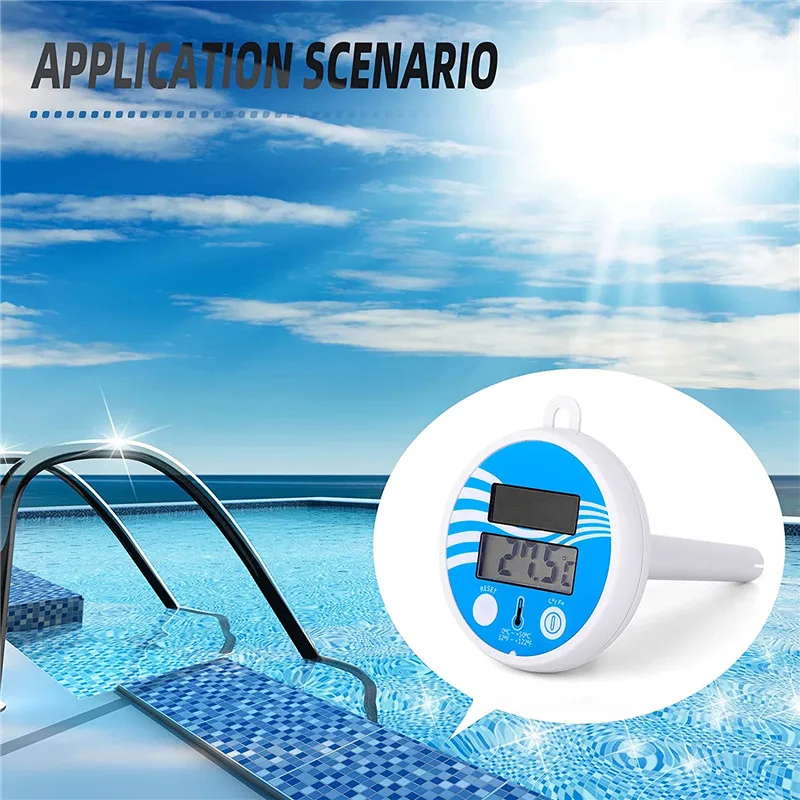This detailed image demonstrates a pool thermometer within a computer-generated outdoor swimming pool setting. The scene highlights a swimming pool with sparkling clear blue water, bordered by charming blue tiles and equipped with handrails for steps leading into the pool. The bright, sunny day is accentuated by a luminous white circle in the upper right corner representing the sun, casting a gleam on the silver handrails. The clear sky and light clouds add to the serene atmosphere. In the upper left corner, the black text "Application Scenario" is prominently displayed. A magnified white bubble showcases a close-up of the pool thermometer, which is white with a blue top, clearly indicating a temperature of 27.5 degrees Celsius – ideal for a warm swim.